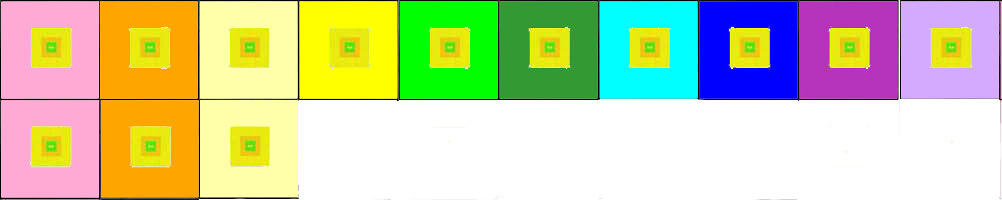The image displays a structured layout of colored square blocks arranged in a single horizontal row and an additional vertical column to the right consisting of three blocks. The main row features ten square blocks, each a different color: pink, orange, light yellow, bright yellow, light green, dark green, light blue, dark blue, dark purple, and light purple. Each of these main squares contains a pattern of nested shapes: a smaller yellow square inside the main square, an even smaller orange square inside the yellow one, and a green circle with a white dot in the center of the orange square. The three-block vertical column to the right repeats the first three colors—pink, orange, and light yellow—and includes the same pattern of nested squares within.